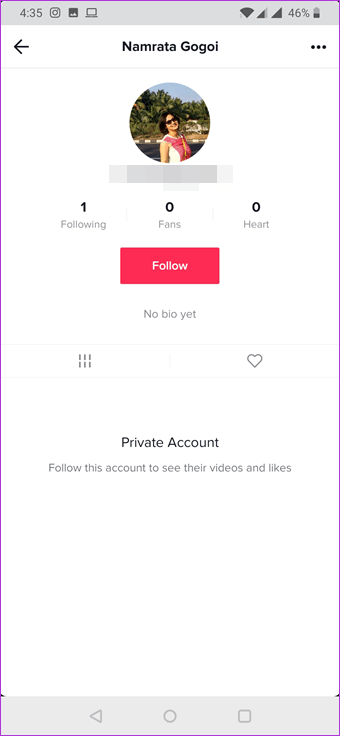This screenshot captures the profile page of a user named Namrata Gogoi. At the top of the screen, positioned below the phone's icon bar, is Namrata's full name. To the left of her name is a back arrow, and on the right is a three-dotted horizontal icon. The profile picture, situated just below the name, features a woman outdoors with trees in the background. She is facing towards the right, turning her head slightly to look at the camera over her right shoulder. Directly beneath the profile picture, there is a redacted section, likely obscuring the user's handle. The profile statistics indicate that Namrata is following one account, has zero fans, and has received zero hearts. At the bottom of the screenshot, a prominent red "Follow" button is displayed, offering an option to follow the user.